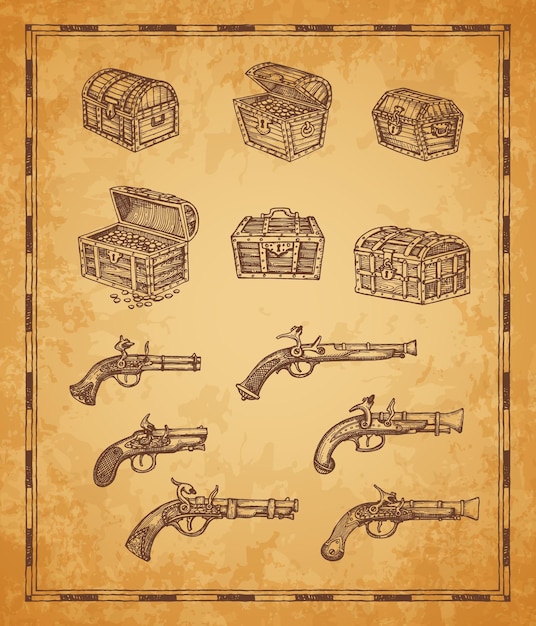This detailed illustration, rendered on aged sepia-colored paper with a black and white alternating bar border, depicts a collection of treasure chests and pistols reminiscent of pirate lore. At the top, six treasure chests are arranged in two rows. To the far left, a completely shut chest contrasts with its neighbor to the right, which is partially open, revealing gleaming pieces of gold. Further right, a locked chest stands firm. In the second row, an almost fully opened chest spills gold, with some coins even scattered on the ground. Adjacent to it, an unlocked yet shut chest sits next to another that is securely locked. Below these chests are six exquisitely detailed, single-shot flintlock pistols with curved handles, reminiscent of the type used in the 1800s or earlier, completing the antique aesthetic of the illustration.